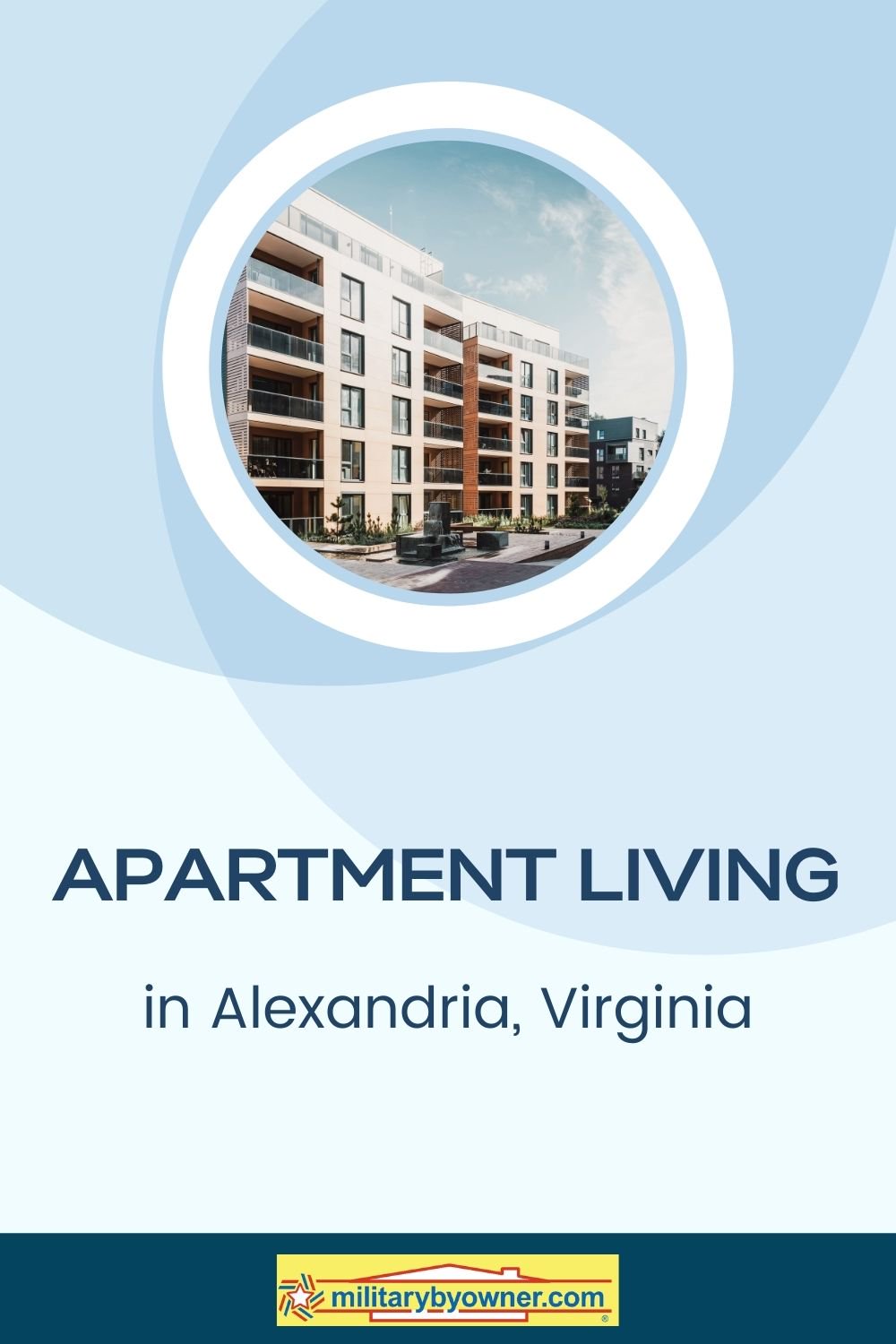The image features a website header and an apartment complex. At the bottom of the image, there is a dark blue bar containing a yellow bar with the outline of a house and two red lines, alongside the text "MilitaryByOwner.com." Above this, in large dark blue letters, it reads "Apartment Living," followed by slightly smaller text that states "in Alexandria, Virginia."

A white circle is prominent in the middle of the image, showing a detailed view of an apartment complex. The building is six stories tall, although the sixth story is set back slightly from the rest. The facade of the building is a creamy white with dark brown, coppery trim. Each apartment has its own balcony, with two adjacent balconies meeting in some areas, while individual corner balconies are also visible. The background features a blue sky filled with numerous clouds. Adjacent to this main apartment building, another building is visible, which appears unrelated to the complex from "MilitaryByOwner.com."